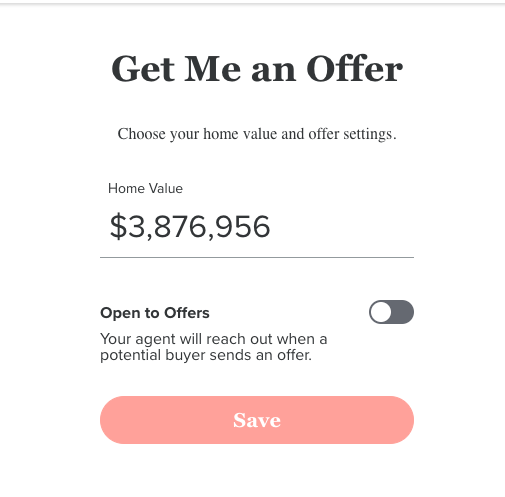The image appears to be a screenshot from a mobile app or web page with a minimalist white background. At the top, there is a section with a prominent, large black font that reads, "Get Me an Offer." Below this header, in slightly smaller gray text, it says, "Choose Your Home Value and Offer Settings."

Beneath this, the text becomes even smaller and thinner, with the gray font displaying the label "Home Value" followed by the large, bold figure "$3,876,956." This value is underlined by an exceptionally thin horizontal line.

Further down, the text "Open to Offers" is displayed in black, accompanied by a toggle switch which looks like a small white circle, indicating it can be clicked to enable or disable the setting. Below this, in small, thin gray text, there is a message that reads, "Your Agent or Reach Out When a Potential Buyer Sends an Offer."

At the bottom of the screen, there is a red cylindrical button with the word "Save" centered in white, uppercase and lowercase letters.